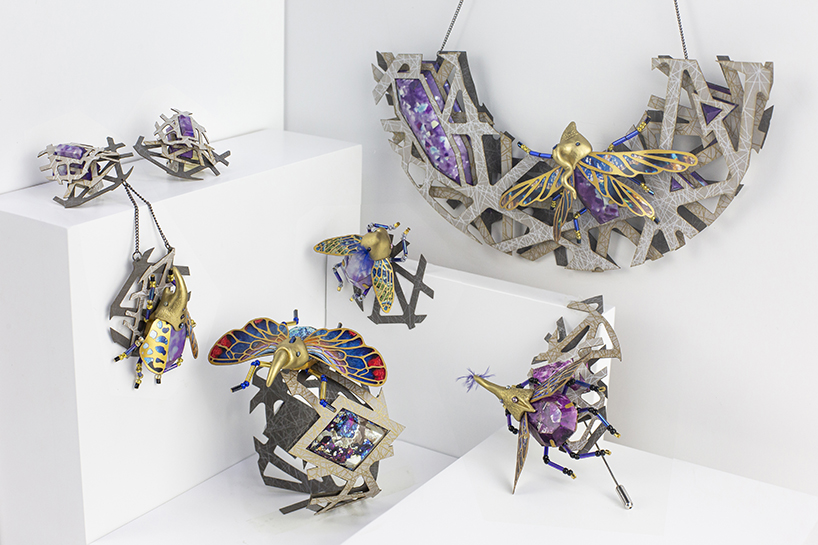This indoor photograph showcases an intricate display of art pieces, primarily in the form of jeweled insect-inspired jewelry crafted from glass, gold, and various colored materials. The background comprises various shades of white, including walls, shelves, and off-white card stock cutouts. The arrangement features six distinct pieces: in the upper right, a hanging artwork resembling a half-moon adorned with purple crystals and a golden dragonfly; on the bottom right, a golden and purple bug, likely a brooch, sitting on a shelf. On a lower shelf, a blue, red, and gold butterfly is placed next to a blue and gold moth. Additional bugs can be seen climbing up a shelf on the far left. The colors evident in this artful ensemble include silver, purple, gold, blue, light blue, red, yellow, and off-white, creating a vibrant and eye-catching display without any accompanying text. The purposeful yet seemingly scattered arrangement of the pieces enhances the visual appeal of this detailed and well-lit indoor scene.